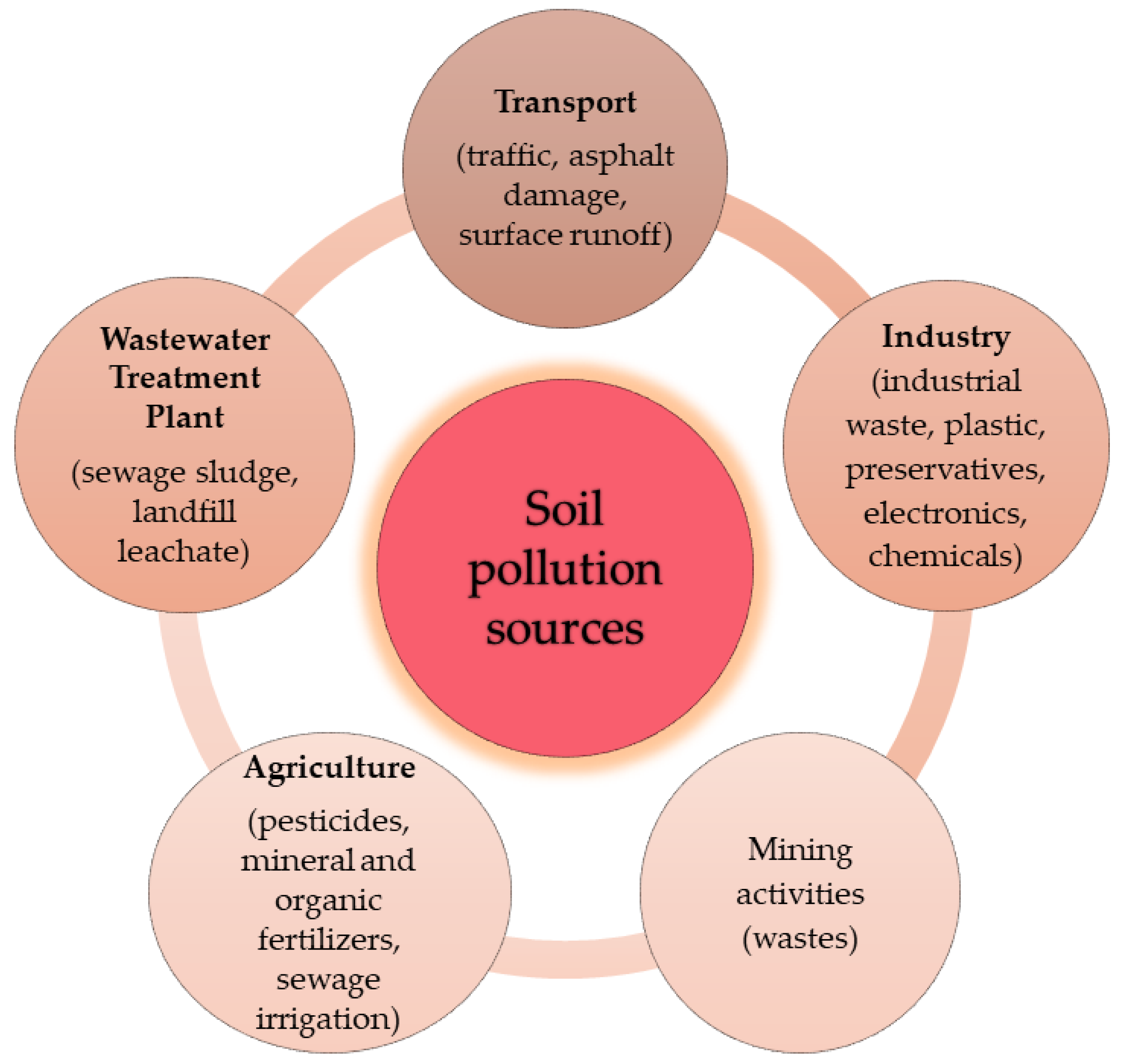The image showcases a detailed diagram of soil pollution sources. At the center of the diagram is a large, salmon-colored circle labeled "Soil Pollution Sources." Surrounding this central circle are five beige circles, each representing a different source of soil pollution. These sources are labeled as follows: 

1. **Transport** (traffic, asphalt damage, surface runoff) — positioned at the top.
2. **Industry** (industrial waste, plastic, preservatives, electronics, chemicals) — to the right.
3. **Mining** (mining activities, waste) — at the bottom.
4. **Agriculture** (pesticides, mineral and organic fertilizers, sewage, irrigation) — to the left.
5. **Wastewater Treatment Plant** (sewage, sludge, landfill leachate) — also to the left, completing the circle around the central focal point.

Each circle's label is written in dark letters, clearly describing the specific pollution sources in detailed subpoints, contributing to an overall very informative visual summary of how various activities contribute to soil pollution.